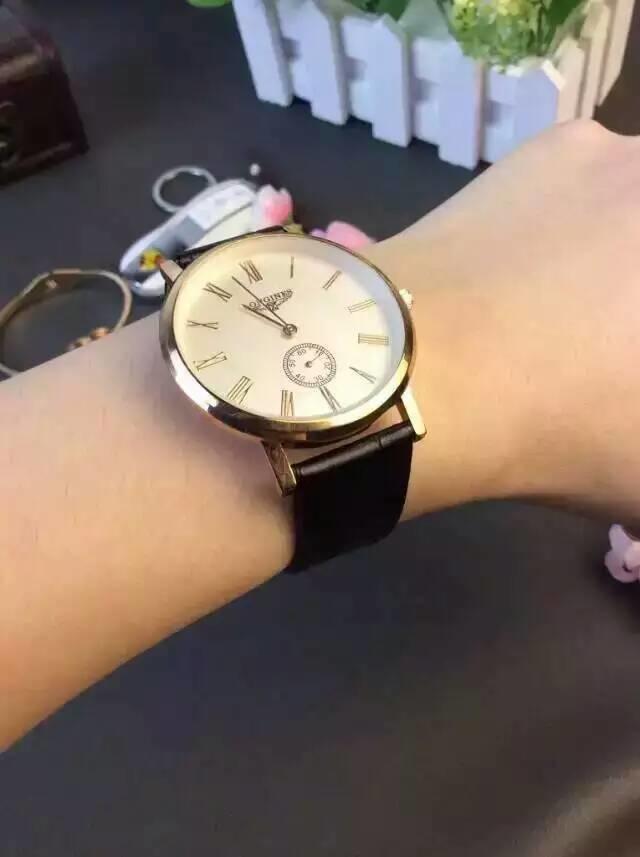This close-up color photograph captures a light-skinned individual's wrist adorned with an elegant analog wristwatch. The watch features a black band and a sophisticated silver housing that encloses the off-white face of the watch. The face is adorned with silver Roman numerals and slender silver hands—the hour hand is pointing at 11 while the minute hand hovers just before the 12, indicating three minutes to 11. A smaller sub-dial in the center displays degrees, marked at intervals from 0 to 60 with fine black hash marks. Surrounding the wrist, the backdrop reveals various objects: a small, decorative white picket fence planter with visible green foliage inside, a white keychain, and a gold bracelet, all situated on a dark grey countertop. Also present, though partially cut off, is a chocolate brown box and vibrant pink flowers, adding a touch of color to the scene.